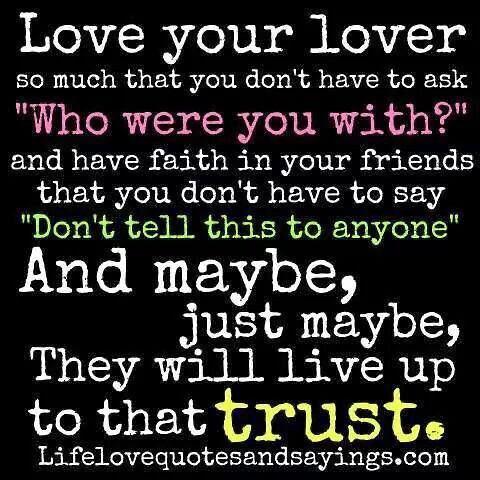The image features a printed saying on a black background with varied lettering colors and sizes for emphasis. At the top in large white letters, it says, "Love your lover so much that you don't have to ask." Directly below that, in pink font, it continues, "Who were you with?" In white lettering, it then reads, "And have faith in your friends that you don't have to say." Further down, "Don't tell this to anyone" is highlighted in yellow. Following this, in white text, it states, "And maybe, just maybe, they will live up to that trust." Here, "trust" is in yellow, as is the period following it. At the very bottom in white, it credits "LiveLoveQuotesAndSayings.com." The use of different colors and font sizes effectively emphasizes key words and phrases throughout the quote.